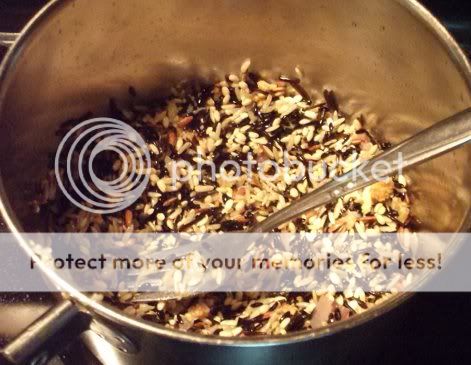The image depicts a somewhat rectangular photograph with a dark palette, primarily composed of browns, yellows, and grays. Central to the picture is a large, round, silver pot, which may appear golden due to the photograph's lighting. The pot contains what looks like rice or cereal at the bottom. Inside the pot, towards the right side, there's a metallic utensil – either a spoon or a fork – angled towards the left.

The photo also contains a faint white band horizontally across it, about a quarter of the way up from the bottom. This band displays black text that is somewhat difficult to read, but it includes the phrase "protect more of your memories for less!" Additionally, there's the Photobucket logo with the words "Photobucket" around the center-left portion of the image.

The overall tone of the image is dark, featuring many shades of brown, tan, gray, black, and gold, suggesting a kitchen setting. The photograph's composition and the positioning of objects emphasize the pot and its contents, as well as the overlaying text and logo.